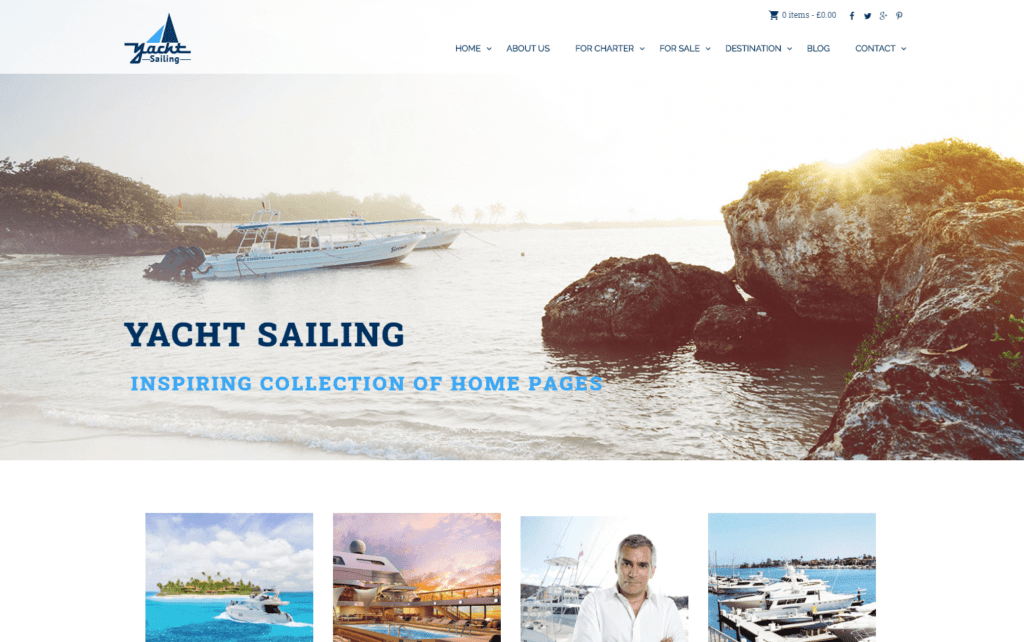At the top left of the image, there's a stylized illustration of a yacht with a sail in light blue and dark blue colors, accompanied by the text "Yacht Sailing." To the right of this illustration, a navigation menu lists the following options: Home, About Us, For Charter, For Sale, Destination, Blog, and Contact. Above the navigation menu, there are social media icons for Facebook, Twitter, and a few other platforms that are not clearly identifiable. Below, a scenic photograph captures a view from the water, showcasing rocks with moss and distant islands. Several yachts are anchored in the water. This image is captioned at the bottom with the text "Yacht Sailing: Inspiring Collection of Home Pages." Beneath this main photo, there are four smaller thumbnails: the first on the left depicts blue water with an island and a yacht sailing in front of it; the next shows the deck of a yacht; the third features a man in a white shirt; and the last thumbnail displays a variety of vessels docked by the water.